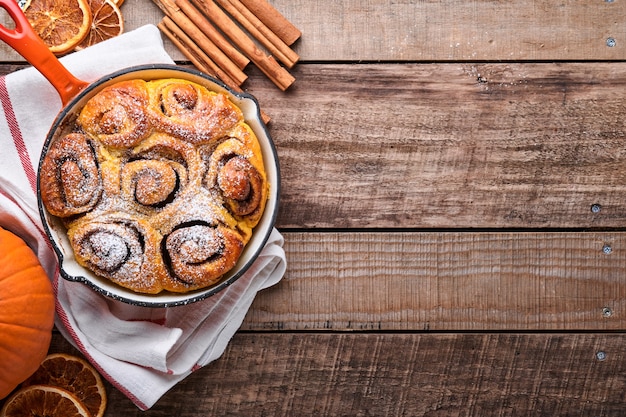A top-down photograph showcases a rustic wooden table with tightly fitted, unfinished boards, still bearing saw marks. In the upper left corner, a white dish towel with a red stripe, folded multiple times, serves as a potholder for a frying pan with an orange handle. Seven freshly baked cinnamon rolls, six around the edge and one in the center, are nestled in the pan, generously dusted with powdered sugar. Complementing the autumnal theme, round orange slices are arranged near the handle and another slice is visible in the bottom left corner. A small pie pumpkin peeks in from the lower left, enhancing the seasonal feel. Scattered near the pan, a few cinnamon sticks add to the rustic, cozy atmosphere.